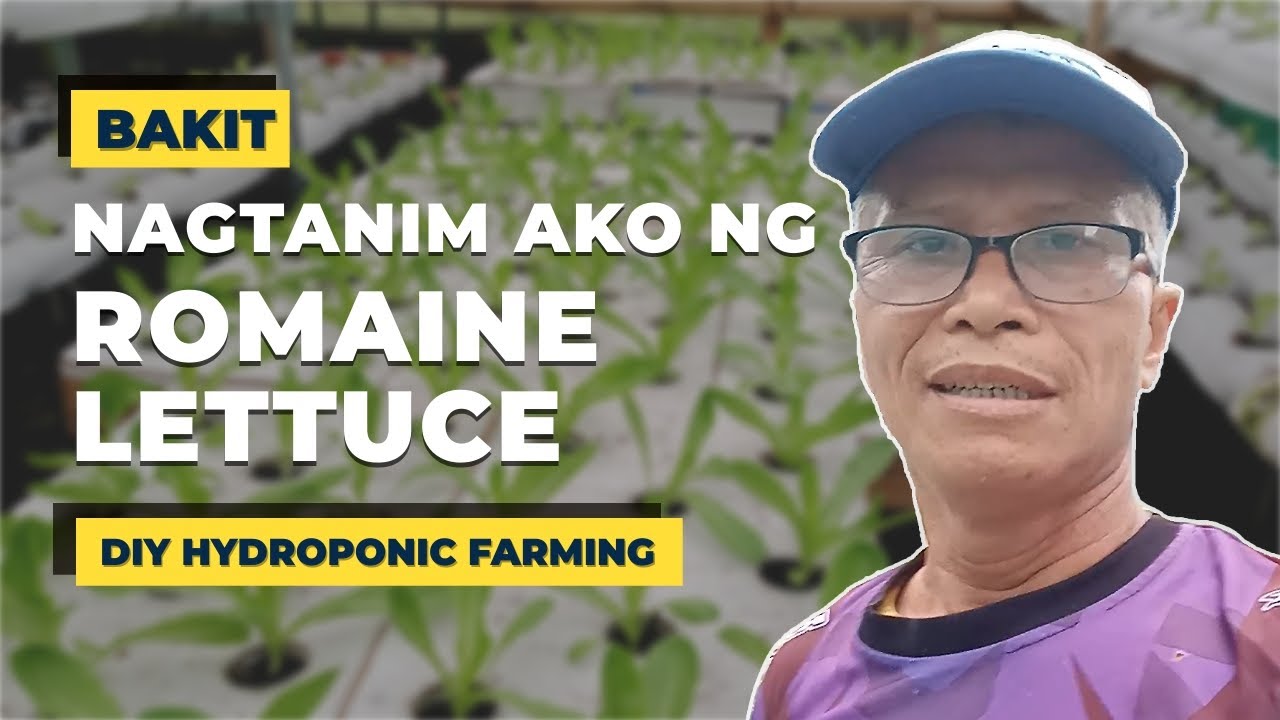The image appears to be an advertisement for DIY hydroponic farming. In the foreground, an older man of likely Asian, possibly Filipino, descent looks directly at the camera. He wears glasses and a blue baseball cap, along with a patterned purple and maroon shirt that has a black neckline. His expression is neutral, with his mouth slightly open. Behind him, the background is blurred but filled with numerous vibrant green plants emerging from white containers, indicative of a hydroponic farming setup.

Prominently displayed on the image is text that reads in black writing with a yellow background: "BAKIT". Beneath it in white text are the words "NAGTANIM AKO NG" followed by "ROMAINE LETTUCE". Another line in black writing on a yellow background reads "DIY HYDROPONIC FARMING". The text and the image together suggest the man is sharing his personal experience or instructions related to hydroponic farming methods, perhaps even as part of an educational online video or presentation.